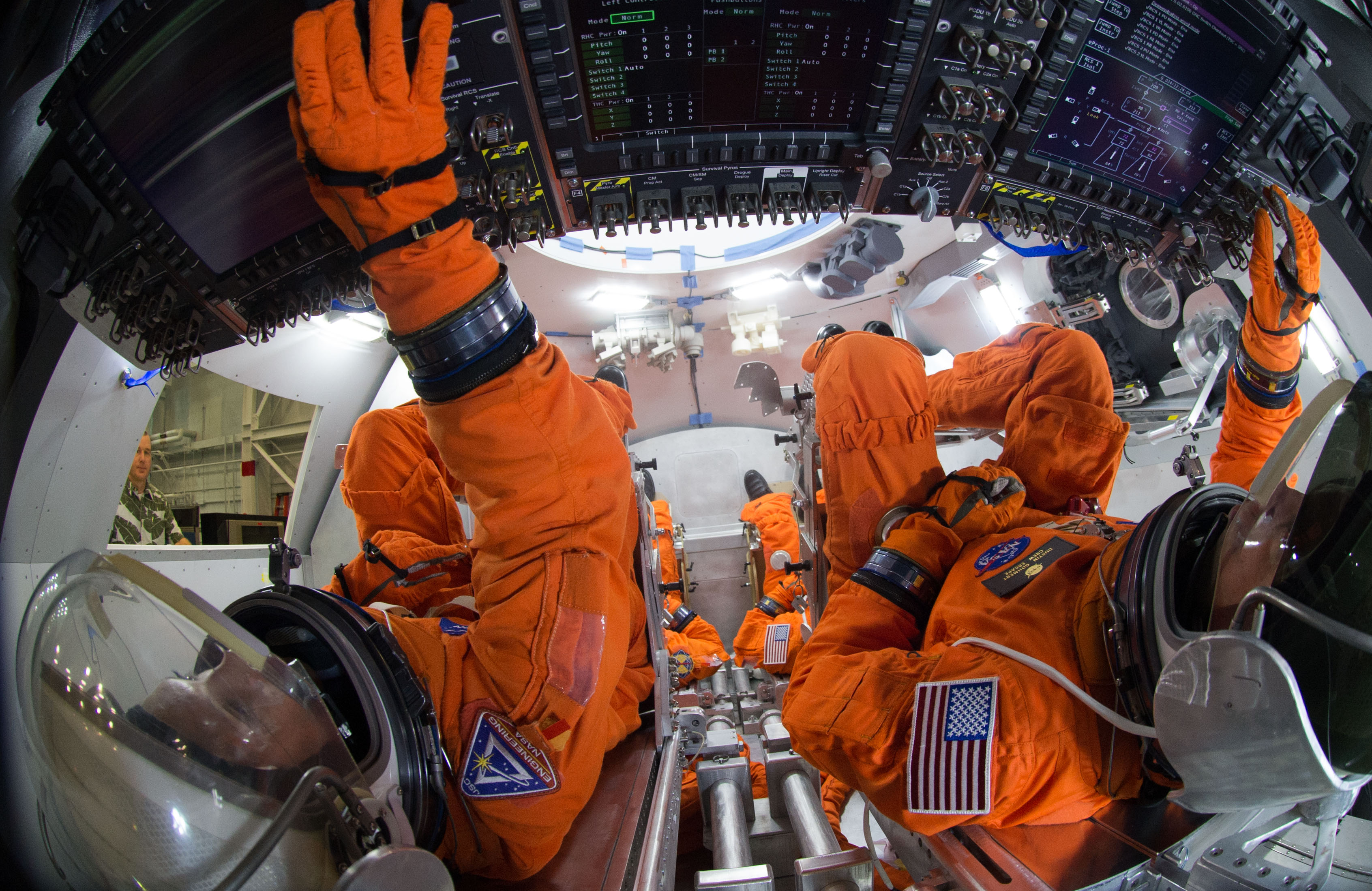The image shows the interior of what appears to be a spacecraft training simulator, featuring two astronauts in the foreground, both adorned in bright orange spacesuits complete with space helmets. These astronauts are seated and strapped into their chairs, focusing intently on a comprehensive instrument panel filled with numerous buttons, screens, knobs, and dials. The photo, taken from a vantage point between their heads, reveals their patches, including the United States flag and NASA emblems, signifying their affiliation. Below this upper level, there are two additional astronauts in identical gear and seating arrangements, emphasizing the multi-tiered structure of the simulator. To the left, visible through a window that suggests an indoor setting, stands a middle-aged Caucasian man in a green and white Hawaiian shirt with leaf patterns, likely overseeing or monitoring the training session. This scene is indicative of astronauts either in training for an upcoming mission or seasoned astronauts refining their skills.